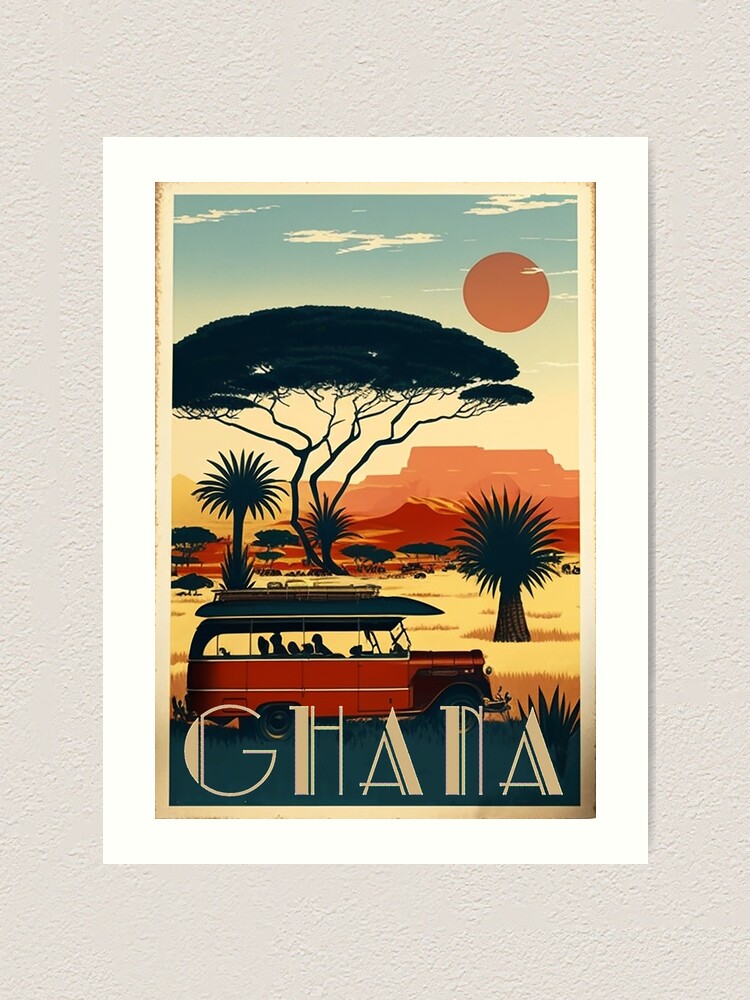This is a detailed depiction of a poster or magazine cover advertising Ghana, rendered in an artistic, vintage Art Deco or nouveau 1920s style. The word "Ghana" is prominently displayed at the bottom in a distinct, fancy uppercase font, with long, art nouveau-style letters in a tannish brown color against a dark bluish background. Behind or just above the letters is an old-fashioned, safari-looking car, possibly red with a bluish roof, absolutely packed with people whose shapes are silhouetted and indistinguishable. The car appears to be driving on a path across the Savannah.

The background showcases the African wilderness with tall yellow grasses and various spiky plants. A large, iconic African yew or savannah tree occupies much of the scene, and you can see plateaus or red-colored mountain rock formations in the distance. A pineapple tree and palm trees further enrich the scene. The muted colors imbue a warm feeling typical of a savannah. The sky above is light blue with sparse clouds and features a soft light orange sun, enhancing the serene, vast landscape.